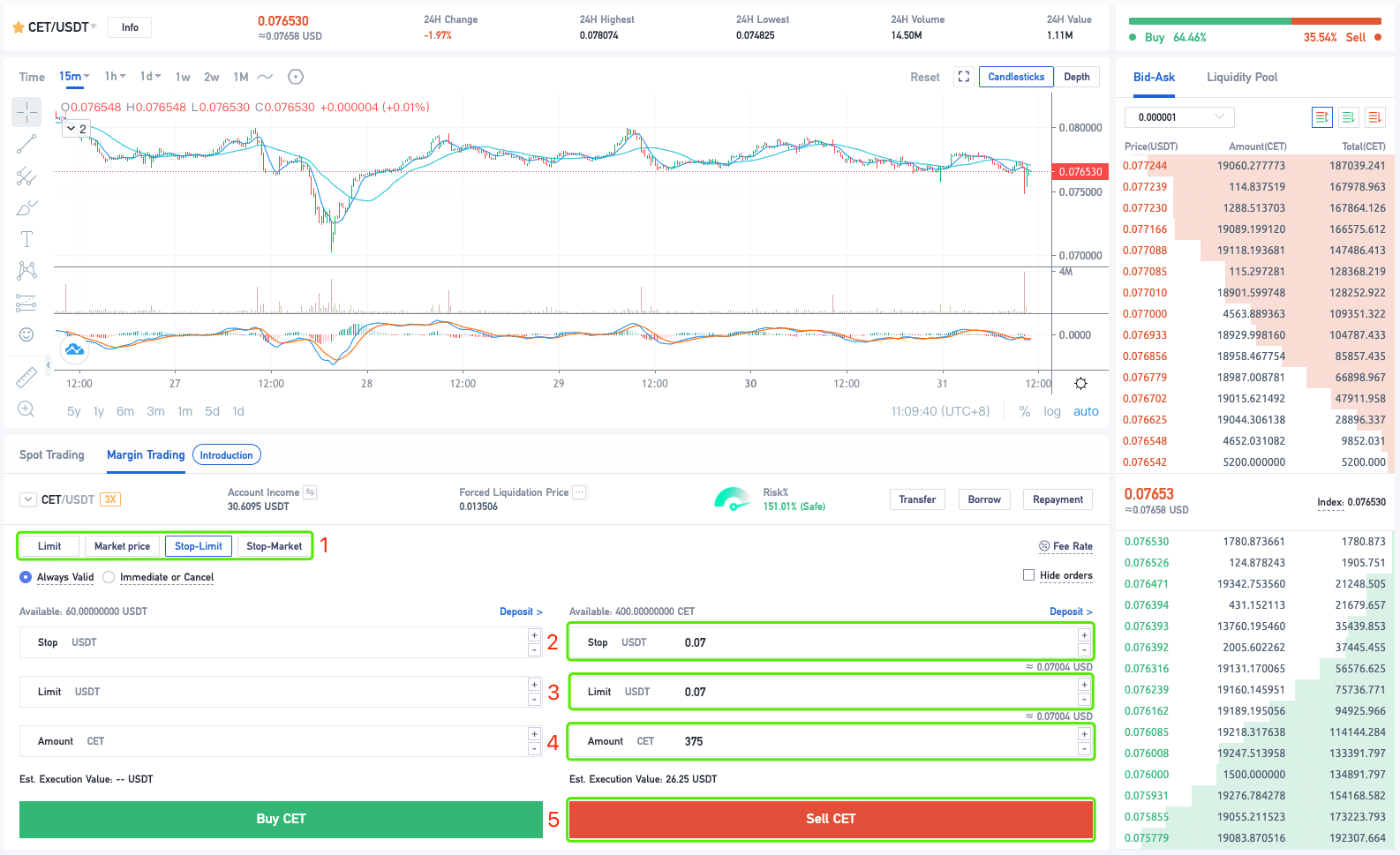The image appears to be a stock-like visual, predominantly displaying a trading platform interface. 

At the top of the screen, a line graph stretches horizontally from left to right, stopping just before the end of the right side. Directly beneath this graph is a central section highlighting "Margin Trading," which is currently selected, contrasting against the "Spot Trading" option visible alongside it.

Towards the right section of the image, there is a vertical list composed of three rows and multiple columns of numbers. This list is color-coded, with red numbers in the top section indicating sell orders and green numbers in the bottom section indicating buy orders.

In the upper left corner of the interface, the trading pair "C-E-T/USDT" is prominently displayed in bold, accompanied by a star symbol located to the left of the text, suggesting it might be favorited or marked for easy access.